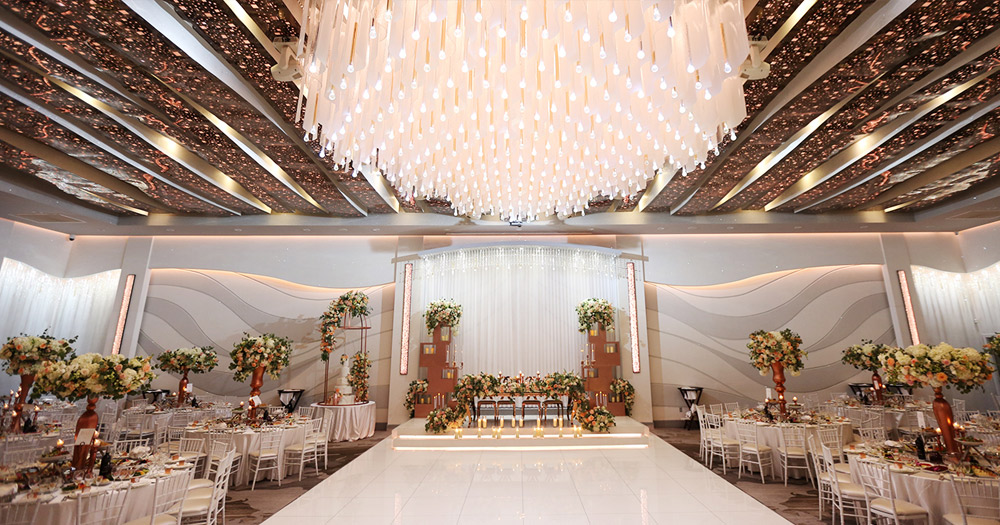The photograph depicts an opulent indoor dining area set up for a wedding reception. Dominating the center of the room is a large, white, stage-like platform adorned with glistening marble tiles. Suspended above the stage is a grand, cylindrical chandelier that cascades down like a shimmering focal point. The ceiling is adorned with fairy lights that twinkle like stars, enhancing the ambiance with a touch of magic. 

In the background, a white altar is decorated with abundant floral arrangements, creating a picturesque focal point. The dining area is flanked on both sides by round, white tables surrounded by matching chairs. Each table features a lavish bronze vase bursting with a mix of white, orange, and green flowers, complemented by lit candles to add a warm glow. The tables are set with plates and cups, meticulously prepared for the celebration.

The left and right sections of the room mirror each other, both transitioning from tiled to carpeted flooring as you move away from the stage. The walls, painted in a subtle gray hue, provide a neutral backdrop that enhances the room's elegance. A pristine white wedding cake, encircled by flowers, sits near the center, promising a delightful conclusion to the festivities.